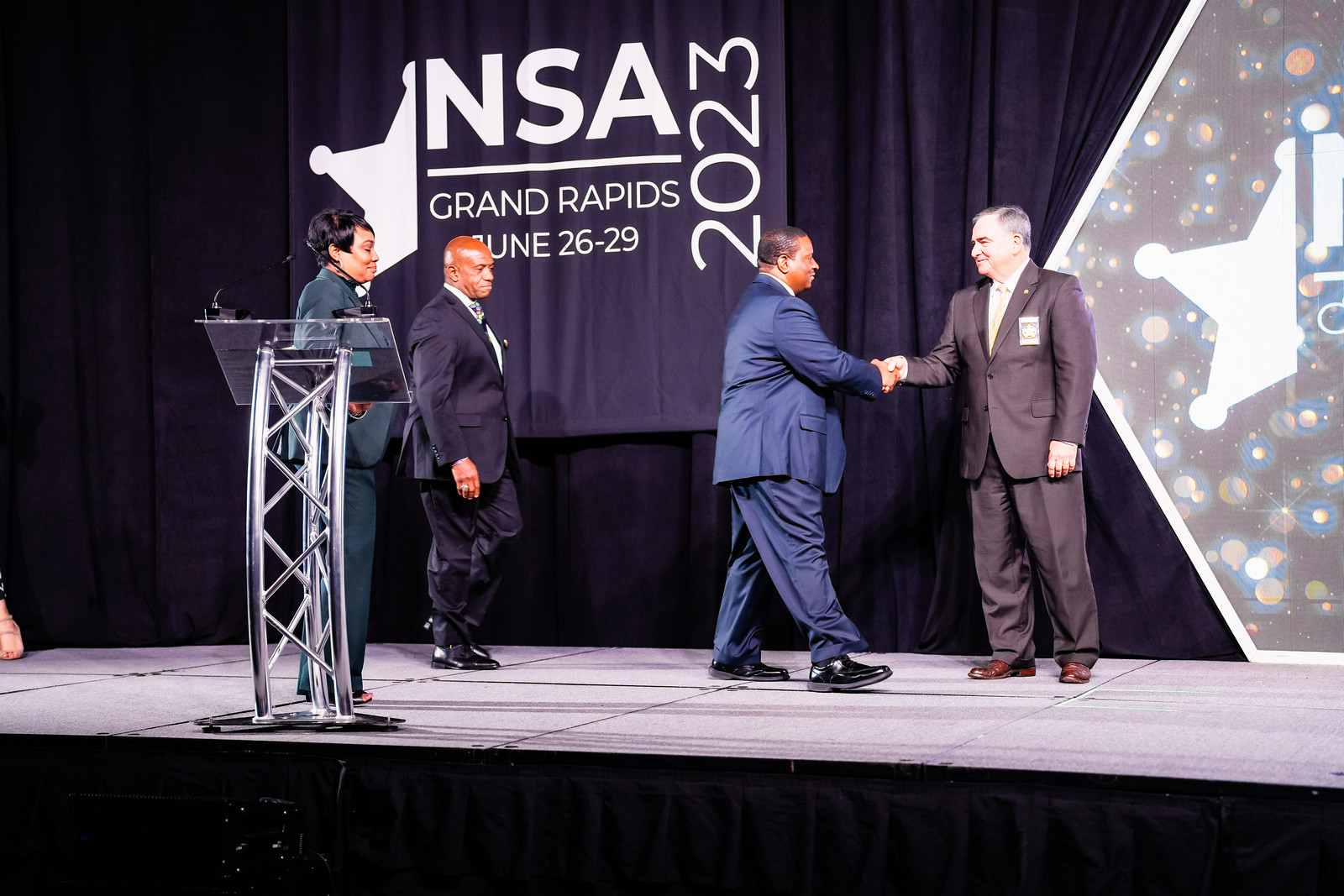On stage at the NSA Grand Rapids awards ceremony, held from June 26 to 29, four individuals are prominently featured. On the right, a white man with gray hair, dressed in a dark blue suit, a white shirt, and a white tie, is sitting and reaching out with his left hand to shake hands with a black man approaching him. This black man, also in a blue suit and black shoes, faces directly towards the seated man, giving a clear side profile view. 

Further back on the left side of the stage, a bald black man in a dark blue suit stands next to a podium with silver supports and a plexiglass top. Beside him is a black woman in a green suit with short black hair, facing towards the right. Hanging behind them is a large, navy blue banner with white text reading "NSA 2023 Grand Rapids, June 26 - 29" alongside a white half-star. The stage features a light gray floor with black lines, and to the far right, there's a section displaying an intricate design resembling microscopic molecules with orange circles and blue lines against a dark backdrop, also featuring a white half-star.